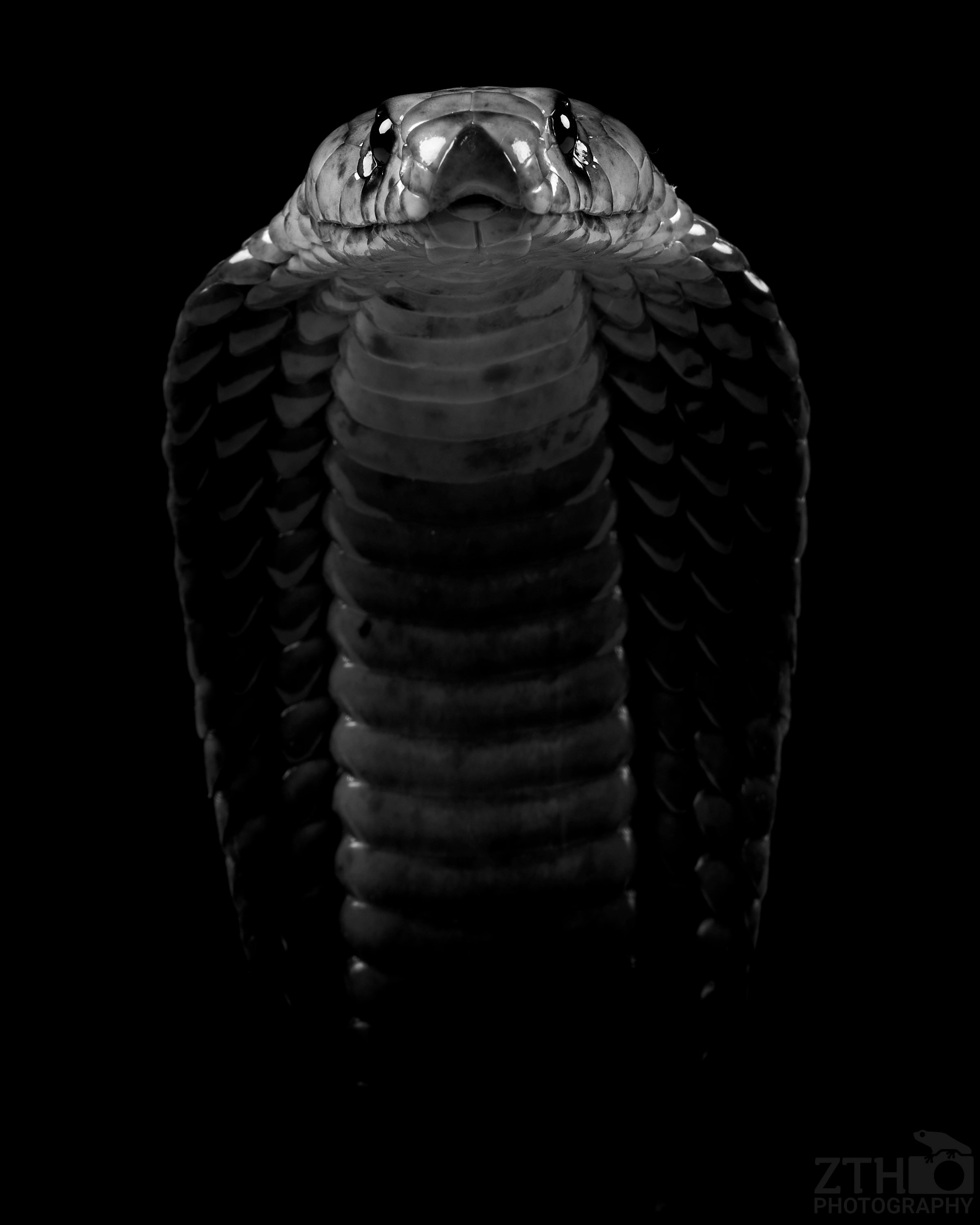This is a highly detailed black and white photograph of a snake, likely a cobra, set against an opaque black background. The image is portrait-style and very zoomed in, showing the snake from the top of its head down to a few inches below what would be considered its neck. The snake's body blends seamlessly into the dark background, creating a mesmerizing fading effect as it disappears into the shadows. The focus of the photograph is on the snake's head, where the interplay of light highlights its reflective, shiny scales. Its eyes, dark with white circles, draw immediate attention, and its mouth is slightly open, adding an intense, almost ominous quality to its gaze. The bottom left or bottom right of the image is marked with the signature "ZTH Photography," ensuring the artist’s acknowledgment. The detailed texture and light reflections strongly suggest that this is a photograph rather than a sketch or painting.